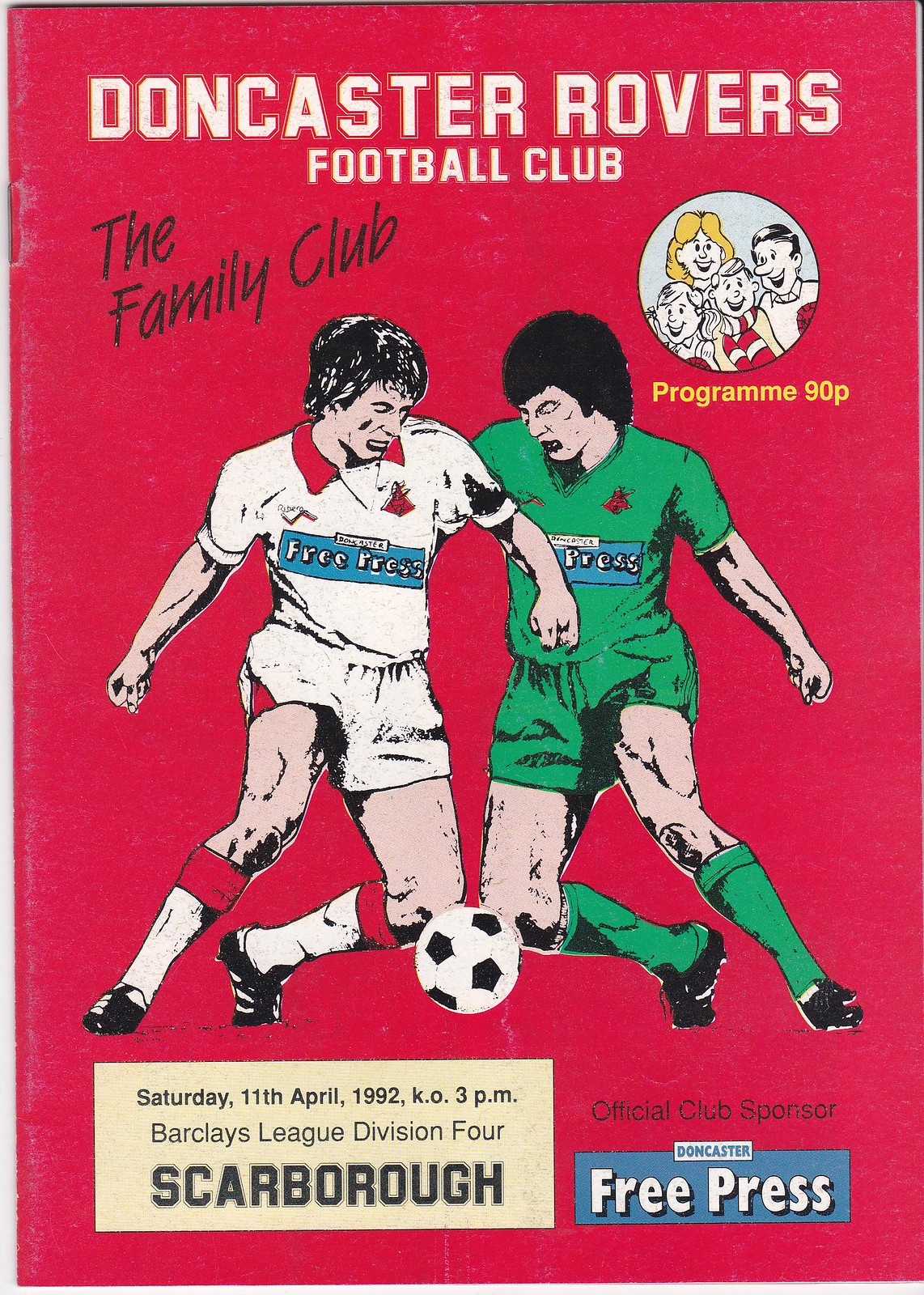The image features the cover of a program for a soccer game with a distinct pinkish-red background. At the top, "Doncaster Rovers Football Club" is prominently displayed in white capital letters. Below this, in black letters, it reads "The Family Club," alongside a simple, cartoon-like illustration of a family—comprising a man, a woman, a boy, and a girl—encircled within a small circle. In the top right quarter, the word "Program" appears in yellow letters, along with its price of "90P." The central illustration depicts two soccer players in action, vying for a soccer ball positioned at the bottom of the image. One player dons a white and red jersey, while the other sports a green jersey. Further visual details show inscriptions on their jerseys that read "Free Press." At the bottom left, within a yellow box, there is information detailing the event: "Saturday, 11th April, 1992, KO, 3 PM,” for a match in the "Barclays League Division 4 against Scarborough." To the right, in black letters, it reads "Official Club Sponsor," with "Doncaster Free Press" showcased below in a blue box.